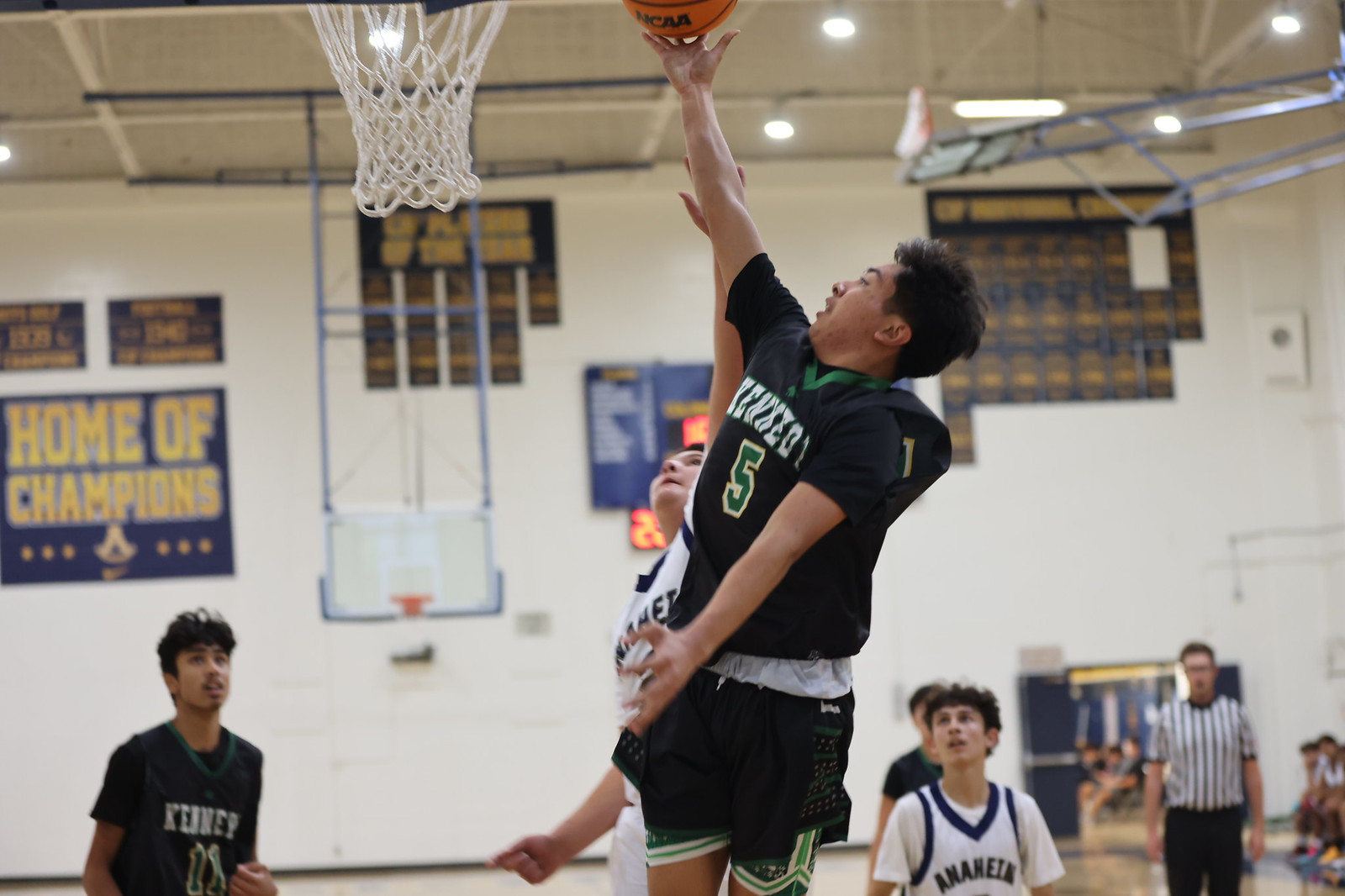The image captures an intense moment of a high school basketball game inside a gymnasium. One player, dressed in a black and green jersey, is leaping into the air, reaching out to perform a layup with an orange NCAA-branded basketball. Simultaneously, a player from the opposing team in white and blue attire is attempting to block the shot. The gym is adorned with signs and banners, including one prominent sign in big yellow text on a blue background stating "Home of Champions." Spectators are visible in the bleachers, and the referee stands nearby, closely observing the action. The scene is set against a backdrop featuring a display of past championships, lending a historic and competitive atmosphere to the game. The lighting from the ceiling illuminates the intense play, capturing the focus and anticipation of everyone present.